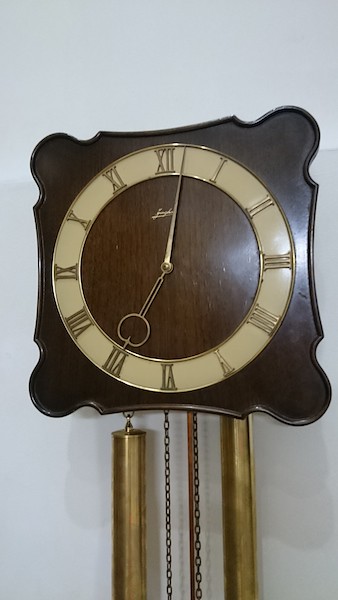The image features a clock mounted on a white wall, highlighted by a prominent brown wooden square backdrop, subtly illuminated to reveal its texture. The clock's central face is circular, marked with numerals from 1 to 12. The minute hand points between the 12 and 1, while the hour hand aligns with 6. 

At the top center of the clock face is a signature, adding a touch of authenticity. The design includes a small metallic bowl at the center, possibly part of the clock's intricate mechanism. Flanking the clock are two substantial cylindrical weights, one on each side, crafted from a metallic copper or bronze material.

Additionally, the clock features two chains running vertically in the middle and on the right, perhaps connected to the weights or internal mechanisms. The entire setup is detailed with numerous small holes, hinting at a complex and possibly vintage clockwork system.